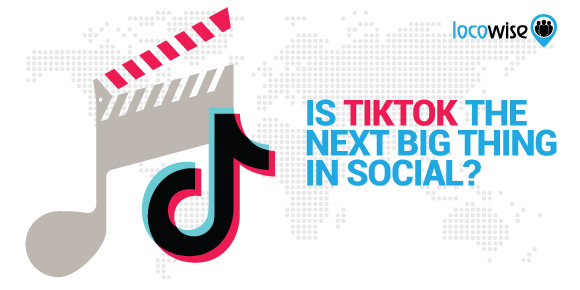Screenshot of a LocoWise Presentation Slide:
   
The image is a screenshot of a presentation slide designed by LocoWise. Located at the top-right corner of the slide is the LocoWise logo, accompanied by a GPS marker icon with a group of people symbol within it. Centrally positioned on the slide is the main title text that reads: "Is TikTok the Next Big Thing in Social?" The text appears in a light blue color, with the exception of the word "TikTok," which is highlighted in red for emphasis. To the left of the text, there is the recognizable TikTok logo, and adjacent to it, a movie clapperboard icon, adding a visual element related to media and entertainment.